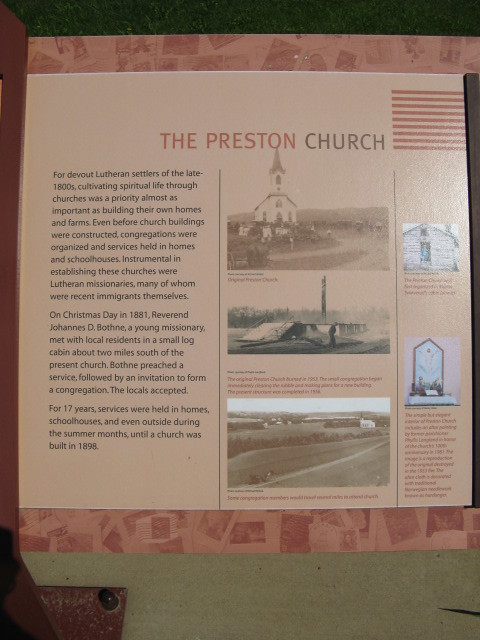This image appears to be a page from an informational book or a placard dedicated to Preston Church, presented in mauve and pink tones. The heading "Preston Church" is prominently centered at the top of the page. Below the heading, there are three sepia and black-and-white photographs showcasing different views of the church during its early years. Along the left side of these photos, a detailed historical narrative explains that for devout Lutheran settlers in the late 1800s, spiritual life through church was a priority nearly as crucial as building homes and farms. Even before physical church buildings existed, congregations organized and held services in homes and schoolhouses. Lutheran missionaries, many of whom were recent immigrants, played a significant role in establishing these churches. The narrative specifically highlights Reverend Johannes D. Bothny, a young missionary who, on Christmas Day in 1881, preached to local residents in a small log cabin located about two miles south of the present church. This service led to the formation of the congregation. For the next 17 years, services were frequently held in homes, schoolhouses, and even outdoors during summer until the construction of the church in 1898. On the right side of the page, two additional photographs depict an old building and what appears to be a mirror or a centerpiece table, accompanied by brief descriptions.